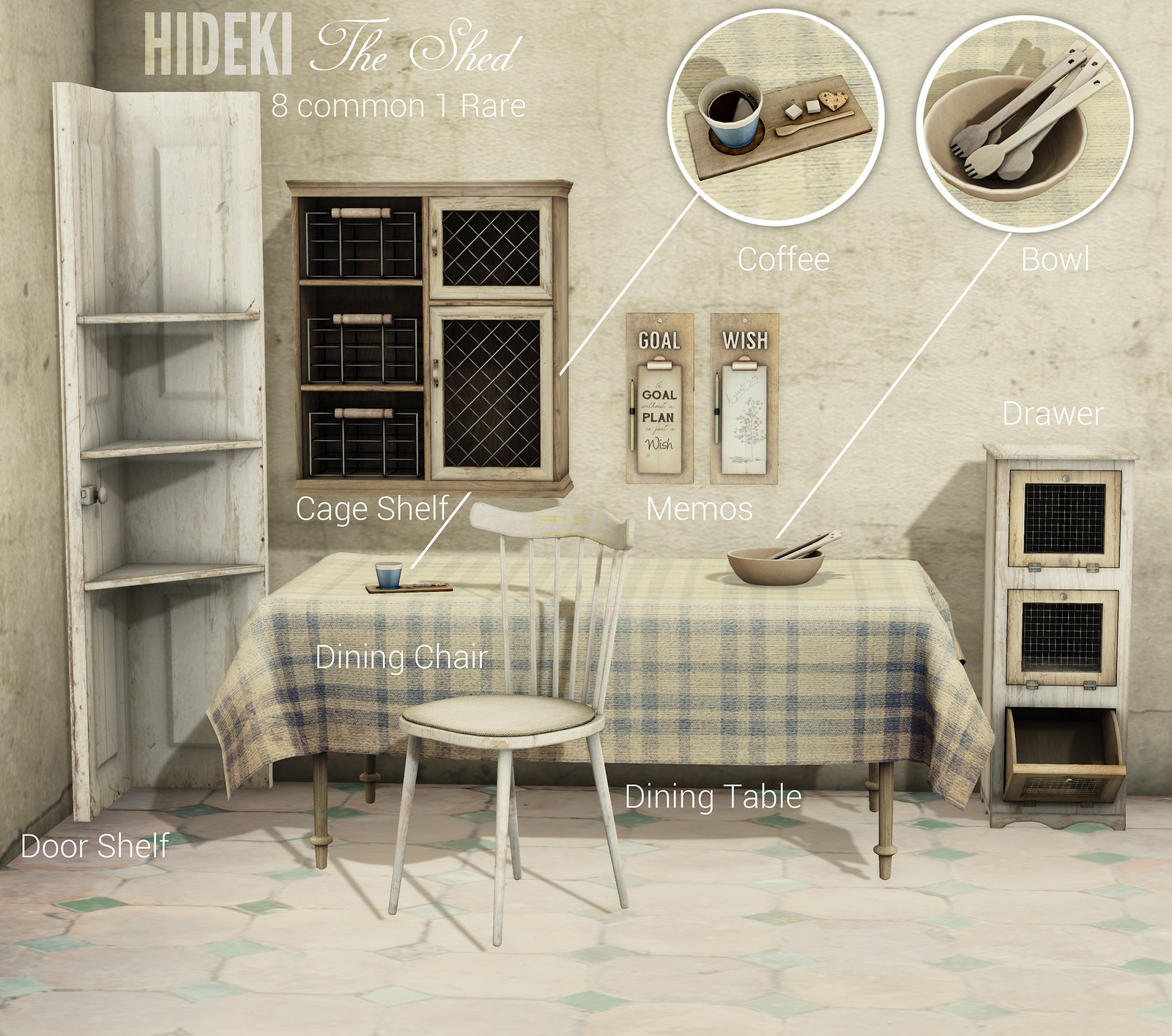The image depicts a rustic dining room with a grey and white wall that appears old and weathered. In the far left corner, there's a unique white corner shelf made from a cut door, featuring three triangular wooden levels. Beside it, a long dining table with thin wooden legs is covered with a wool tablecloth in a blue and yellow checkered pattern, complemented by a white chair in front. On the table, there's a small blue cup. Above the table, a cage shelf is mounted on the wall, comprising three shelves with baskets and two additional caged sections. The wall displays several clipboards with memos, one reading "Gold Plan" and another "Wish." The upper part of the image has text that says "Hide the key, the shed, 8 common, 1 rare." Additionally, zoomed-in images in the top right corner highlight a bowl with cutlery and a coffee cup on a piece of wood with a spoon and some sugar, pointing out details within the room. Alongside the dining table, there's a horizontal set of drawers adding to the room's farmhouse ambiance.